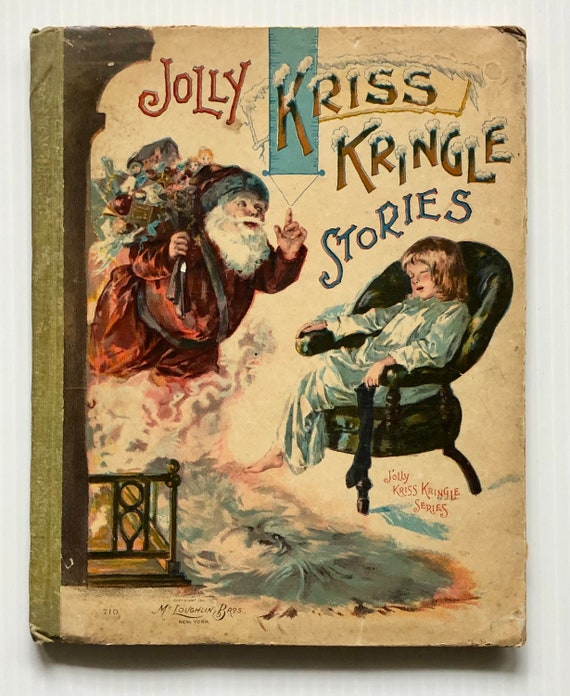The cover of this old, vintage children's storybook titled "Jolly Kris Kringle Stories" features a worn, beige background. Dominating the left side is an illustration of Santa Claus, or Kris Kringle, dressed in his iconic red suit with a large white beard and a sack of toys slung over his back. The design gives a sense that Santa may have emerged from a fireplace, blending slightly into the paper.

On the right side, there is a young child with brown hair, wearing a light turquoise nightgown, sitting in a padded armchair, depicted as if they have waited up to catch a glimpse of Santa. The child is in pajamas and appears to be slipping into sleep. The chair is black with cushion padding on the seat and back. Below the word "Stories," which is printed in blue text, the child rests on a light-colored rug. 

The book's title is displayed prominently: "Jolly Kris Kringle" is written with the word "Jolly" in bright red and "Kris Kringle" in dark orange text adorned with snow on each letter.